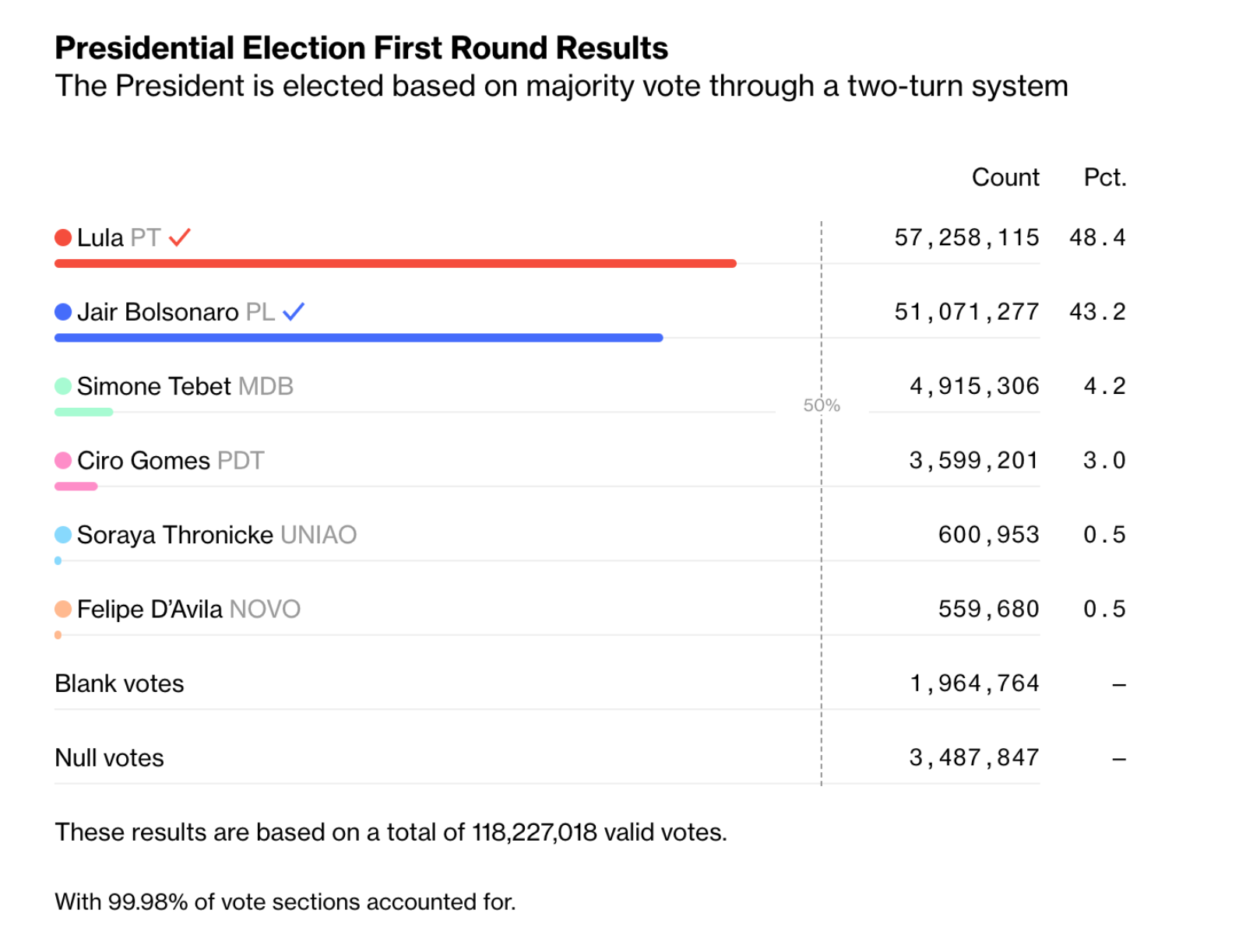The image displays a detailed results screen on a news website for the first round of the presidential election. At the top, in bold black letters, it reads "Presidential Election First Round Results." Beneath this, there's a note indicating that the president is elected based on a majority vote using a two-turn system.

On the left-hand side of the screen, the names of the candidates are listed vertically. To the right of the names, there's a column labeled "Count," which shows the number of votes each candidate received. Further right, another column labeled "Percent" displays the percentage of total votes each candidate garnered. 

At the top of the candidates' list is Lula, representing the PT party, marked with a red check mark. A red bar beneath his name extends almost to the edge of the column, reflecting his vote count and percentage. Lula has received 57,258,115 votes, translating to 48.4% of the total votes.

Below Lula, the next candidate listed is Jair Bolsonaro from the PL party. His vote count is represented by a blue bar, which is significantly shorter than Lula's red bar. Bolsonaro has garnered 51,071,277 votes, equating to 43.2% of the total votes.

The candidates and their respective vote counts and percentages continue to be listed down the page. A dashed gray line runs vertically between the candidate names and the columns for vote count and percentage, indicating the 50% mark needed for a candidate to win outright in the first round.